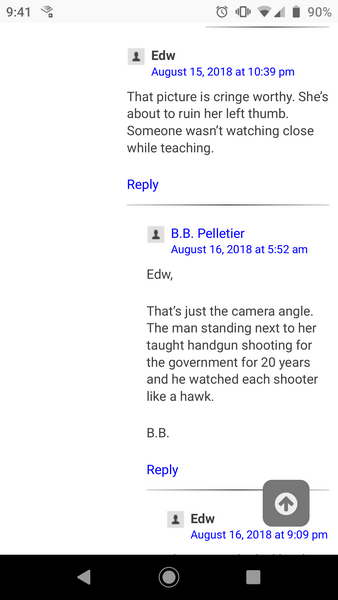The image depicts a smartphone screen displaying a conversation. At the top left corner, the time reads "9:41," and to the right, standard icons are visible: the phone signal icon, a clock icon, an icon resembling a rectangle with three lines extending from it, the Wi-Fi signal icon, and the battery icon showing 90% charge.

The conversation involves two participants, identified as "EDW" and "BBB.B Pelletier," both of whom have default avatars. "EDW" sent a message on August 15, 2018, at 10:39 PM, stating: "That picture is cringeworthy, she's about to ruin her left thumb. Someone wasn't watching closely while teaching."

A reply from "BBB.B Pelletier" follows, dated August 16, 2018, at 5:52 AM. Pelletier responds: "EDW, that's just the camera angle. The man standing next to her has been teaching handgun shooting for the government for 20 years and watches each shooter like a hawk."

There is a further reply from "EDW," dated August 16, 2018, at 9:09 PM, but the content of this reply is not visible in the image.

At the bottom of the screen, navigation buttons are visible: the back button, the home button, and the overview (square) button.